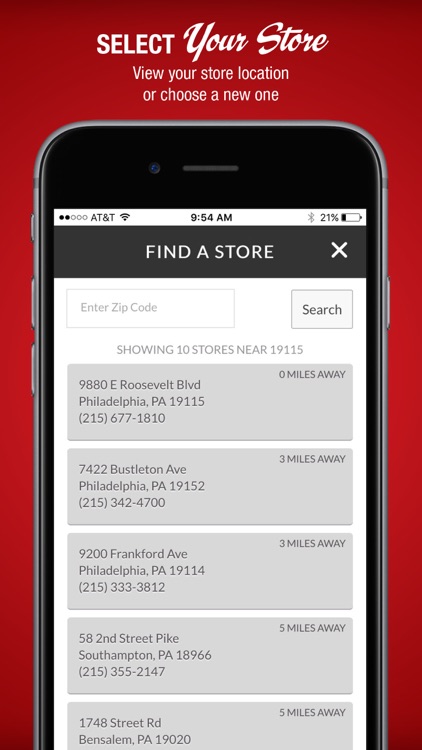A close-up screenshot of a digital interface displays a mobile phone within the interface. At the top of the screen, there is a bold red banner with white text reading "Select Your Store." Below, in smaller white text, it instructs users to "View your store location or choose a new one." Central to the image is a detailed representation of a mobile phone screen. 

In the phone's status bar, the upper-left corner displays the cellular signal strength from AT&T, indicating a weak signal with only 2 out of 5 dots filled. Adjacent to this, a Wi-Fi icon signifies connection, followed by the current time, which is 9:54 AM. Further right, a Bluetooth icon is visible, and next to it, a battery icon showing 21% battery remaining.

Beneath the status bar, a prominent black banner features the command "Find a store," accompanied by a search box where users can enter a zip code for location-based results. Below this banner, the text announces, "Showing 10 stores near 19115," with a list of approximately 5 available store results displayed underneath.